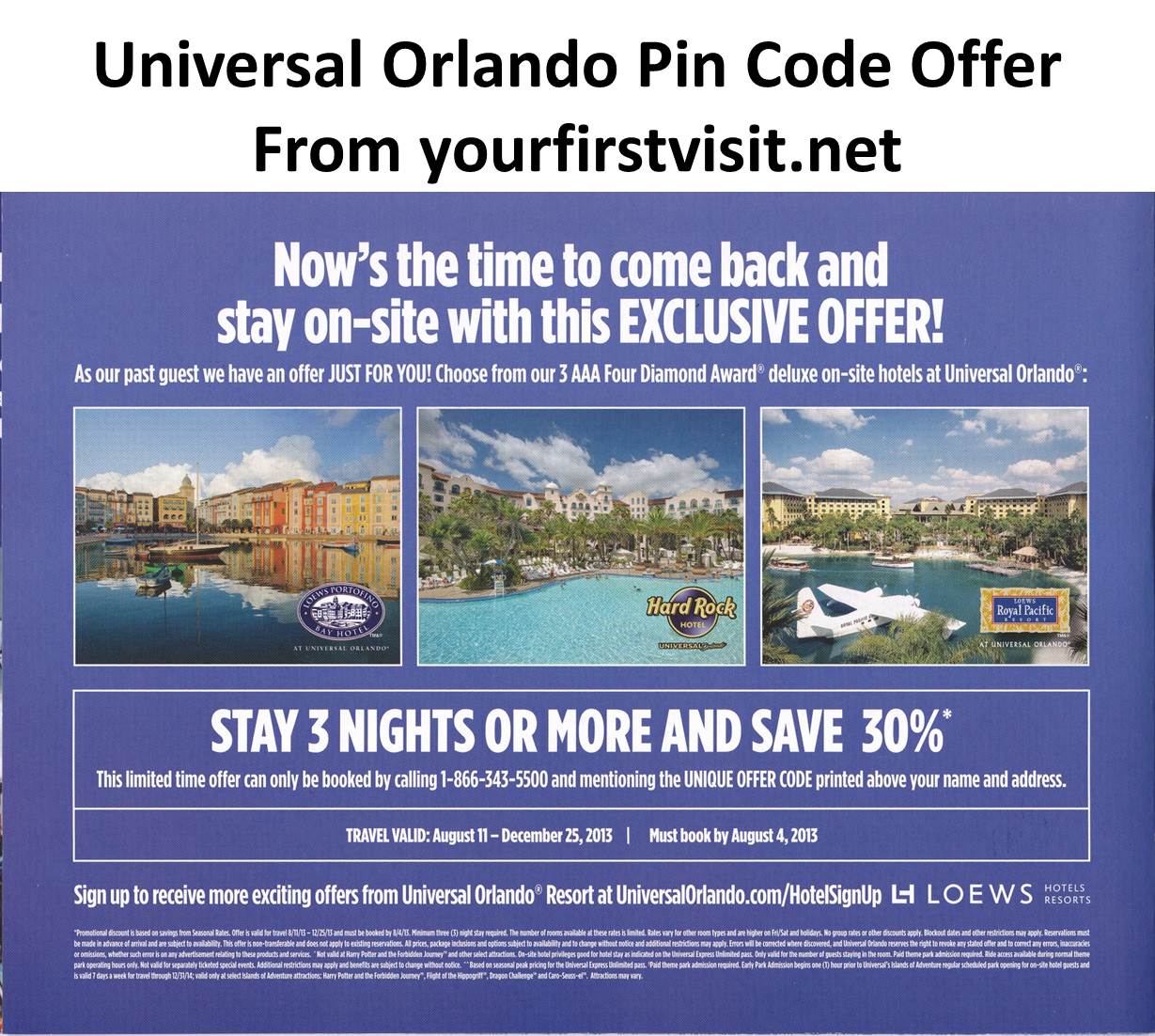### Detailed Caption for Promotional Material Image

The image presents a digital promotional material from Universal Orlando, specifically an offer originating from YourFirstVisit.net. The top section of the image features black text on a clean white background that reads: "Universal Orlando Pin Code Offer from YourFirstVisit.net." Directly beneath this text, a blue box occupies the majority of the image, framed against the white background.

Within the blue box, the central message is prominently displayed. The text encourages previous guests to take advantage of an exclusive deal, stating: "Now's the time to come back and stay on-site with this exclusive offer. As our past guests, we have an offer JUST FOR YOU." Here, "JUST FOR YOU" is emphasized in all capital letters to capture attention.

The promotional material then introduces three AAA Four Diamond Award deluxe onsite hotels at Universal Orlando with thumbnail images for visual appeal. The central thumbnail features Hard Rock Hotel, flanked by thumbnails of two other luxury resorts.

Below these thumbnails, the promotion continues with a compelling offer: "Stay three nights or more and save 30%." It further details that this limited-time offer can only be availed by calling a provided phone number and mentioning a unique offer code, which is printed above the recipient's name and address. The promotion includes validity dates and stipulates that bookings must be completed by August 4th, 2013, indicating that this is a past advertisement.